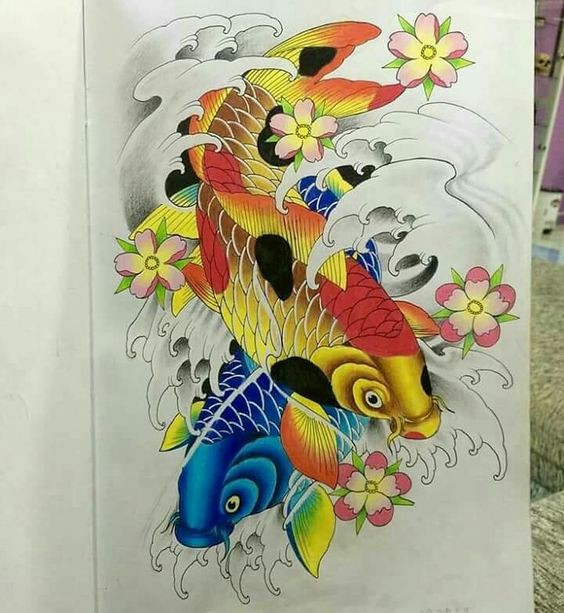This image features a meticulously colored sketch or possibly a page from a pre-drawn coloring book. The artwork vividly depicts an enchanting koi pond, teeming with brilliantly hued koi fish, rendered in striking reds, blues, and greens. The vibrant scene is accentuated by an abundance of detailed flowers and dynamic white waves, evoking the essence of a lively aquatic habitat. The intricate coloring technique remains ambiguous, suggesting either colored pencils or perhaps watercolors as the medium. The piece has been photographed against a neutral gray couch backdrop, which supports the paper but does not distract from the art itself. There is no visible artist’s signature on the piece.